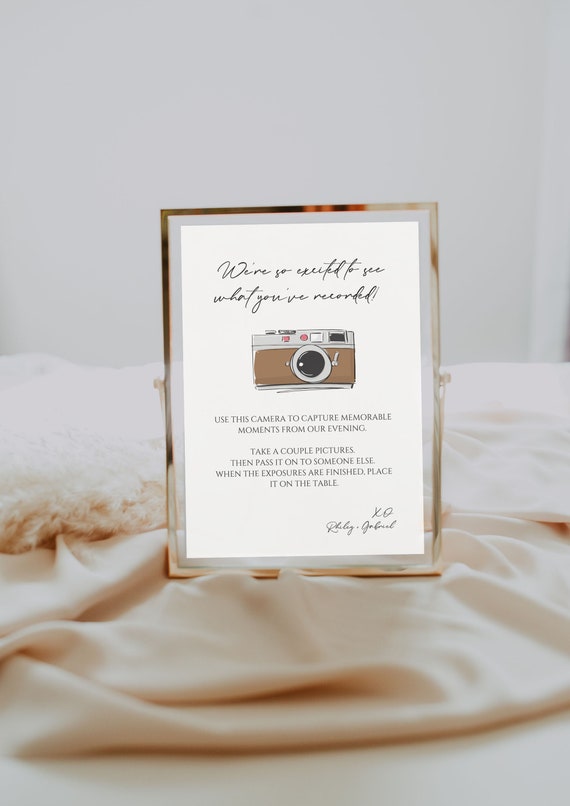The image is an elegant wedding tabletop display featuring a framed note card. The background showcases a white wall adorned with a gold silk-colored fabric and a white fuzzy blanket. At the center of the composition is a gold metal frame housing a white paper-like card. The card presents a hand-drawn, vintage-style camera rendered with colored pencils. The camera, featuring a brown wood-finished body and silver top with a prominent lens, viewfinder, flash, and a small red light, exudes an old-fashioned charm. The text on the note reads: "We're so excited to see what you've recorded." Below the camera, the instructions continue: "Use this camera to capture memorable moments from our evening. Take a couple pictures and pass it on to someone else. When the exposures are finished, place it on the table." In the bottom right corner, there are affectionate initials, "XO," symbolizing the couple's gratitude and love.